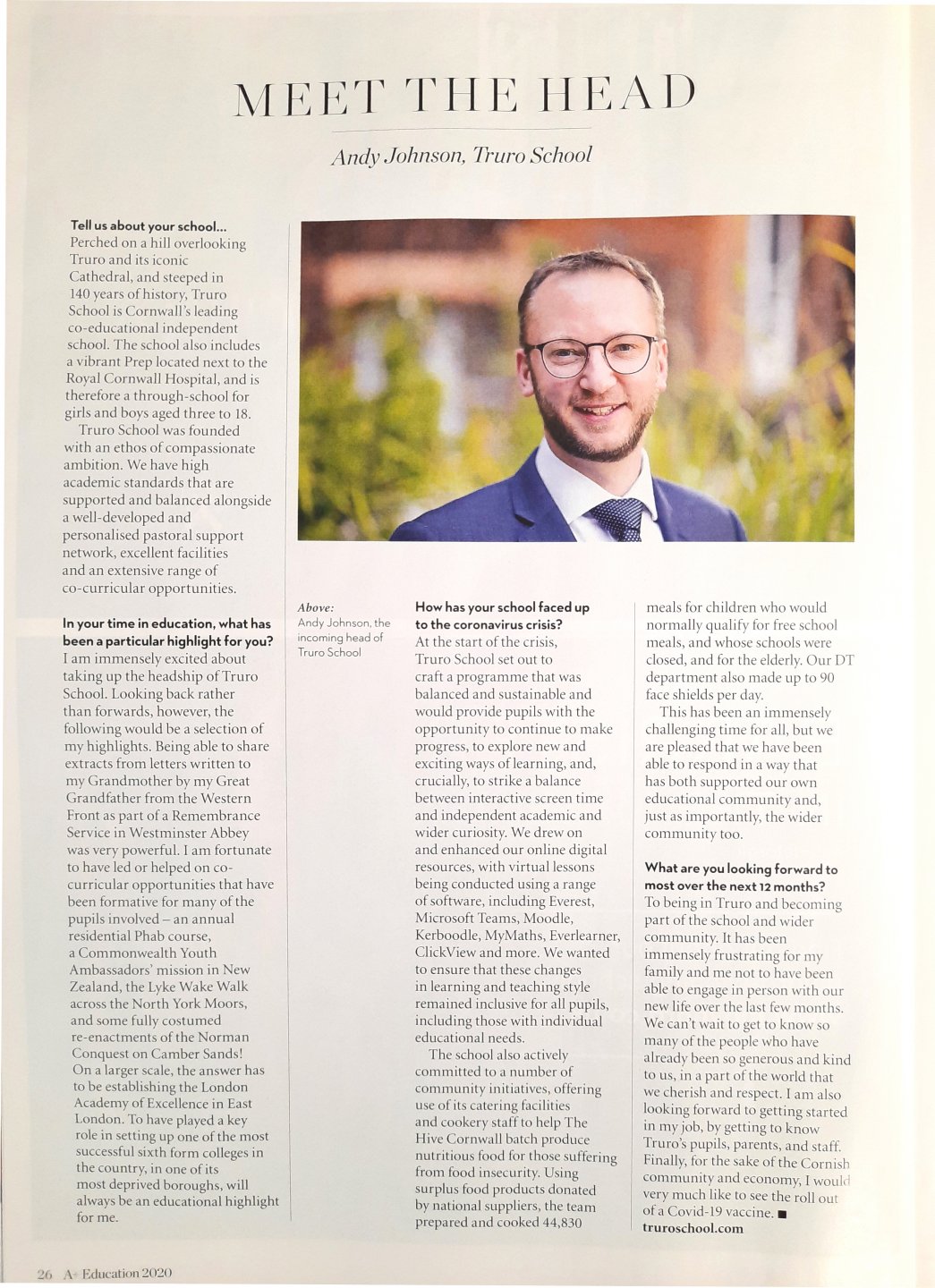The image features a visually appealing magazine article set against a light purple background. The headline reads "Meet the Head," underlined for emphasis. The centerpiece of the article is a large, vibrant photograph of Andy Johnson, who is described as a "true rose ghoul." 

Mr. Johnson appears cheerful and welcoming, with light-colored hair, a pair of glasses, and a neatly trimmed beard. He is dressed in a blue suit paired with a blue tie and a crisp white shirt, projecting a professional yet approachable demeanor.

The article begins with a prompt, "Tell us about your school," followed by several paragraphs where Mr. Johnson elaborates on the institution he leads. A highlighted section draws extra attention to important details, while a central text box provides additional insights about Mr. Johnson. 

There are four distinct columns that delve further into various aspects of his experiences and philosophies. The layout concludes with a small black box accompanied by some final remarks in black print. In essence, the article paints a well-rounded and positive portrait of Andy Johnson, portraying him as a dedicated and joyful head of the school who thoroughly enjoys his responsibilities.